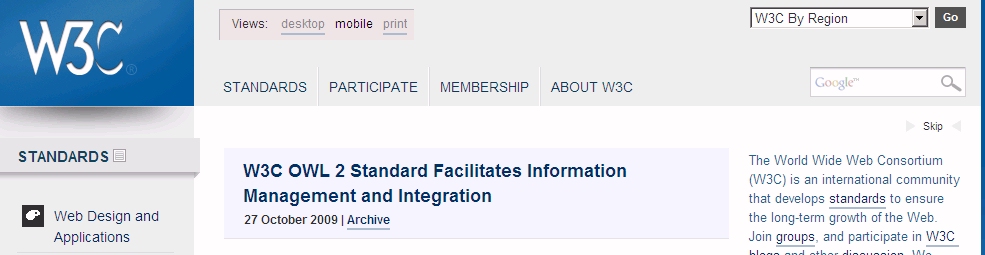The image is a screenshot from the mobile section of the W3C website. The top portion features a deep blue background on the left with the stylized "W3C" logo, which includes a registered trademark symbol. To the right of the logo, a gray navigation bar displays options for "Desktop," "Mobile," and "Print," with "Mobile" highlighted and "Desktop" and "Print" underlined.

Further to the right, there is a search box labeled "W3C by region" with a dropdown menu and a "Go" button featuring a dark gray background and white lettering. Below this navigation bar, there are blue hyperlinks for "Standards," "Participate," "Membership," and "About W3C." Adjacent to these hyperlinks is a search bar with a magnifying glass icon, which presumably connects to Google search functionality.

In the main content area, on the left side, there is a section titled "Standards" in blue text, accompanied by an icon of a notepad. Adjacent to this, the text "Web Design and Applications" appears. Below this section to the left, there is a black box containing a color palette icon with a white center. To the right of this, text reads: “W3C L2 Standard Facilities Information Management and Integration 27 October 2009,” with "Archive" written in blue text indicating it's a clickable link. The "W3C" section title is also in blue, signifying clickable content. On the far right, there is a brief description of the World Wide Web Consortium.

This caption provides a detailed and organized description of the content and layout of the screenshot, ensuring clarity and coherence.